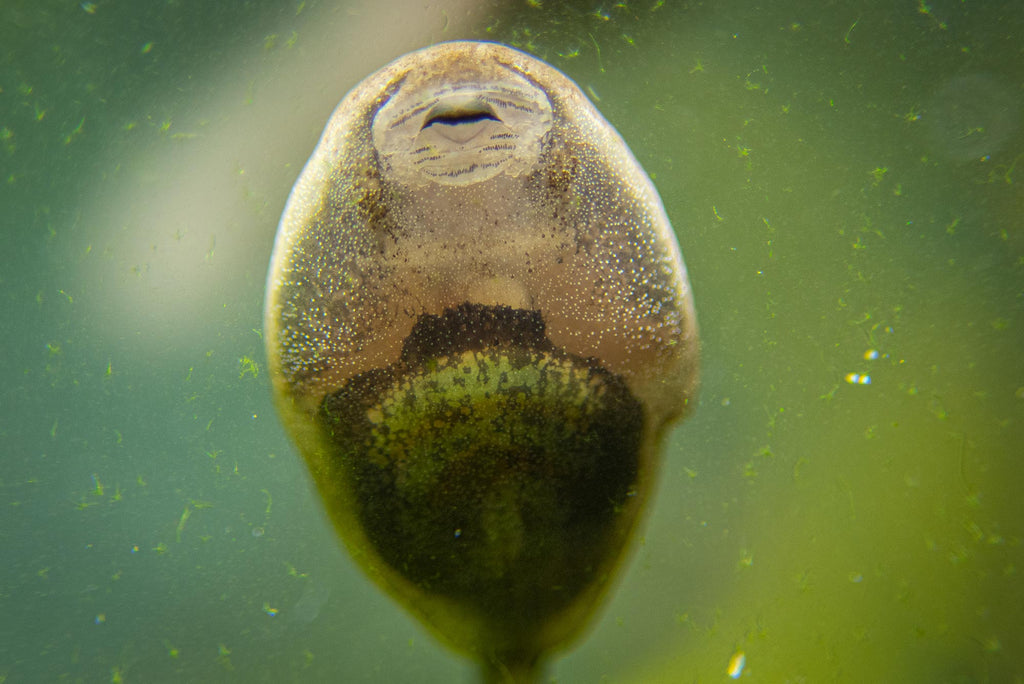The image features a microscopic view of an organism that appears almost elliptical or like the closed bud of a flower, positioned vertically with what seems to be a small stem emerging from its lower end. The organism is distinctly divided into two halves: the upper half is light brown with an eye-like structure in the middle, surrounded by many white dots and intricate black lines. The lower half is green, with darker areas towards the center and the presence of some black markings. Surrounding the organism, the background is blurred and contains numerous tiny, green floating particles. The right side of the background predominantly displays lighter green shades, while the left transitions from a bluish tint at the bottom to darker green towards the top, intersected by a diagonal white line and various small white lights. The overall scene resembles an underwater environment with floating debris, giving it a fuzzy, dream-like appearance.